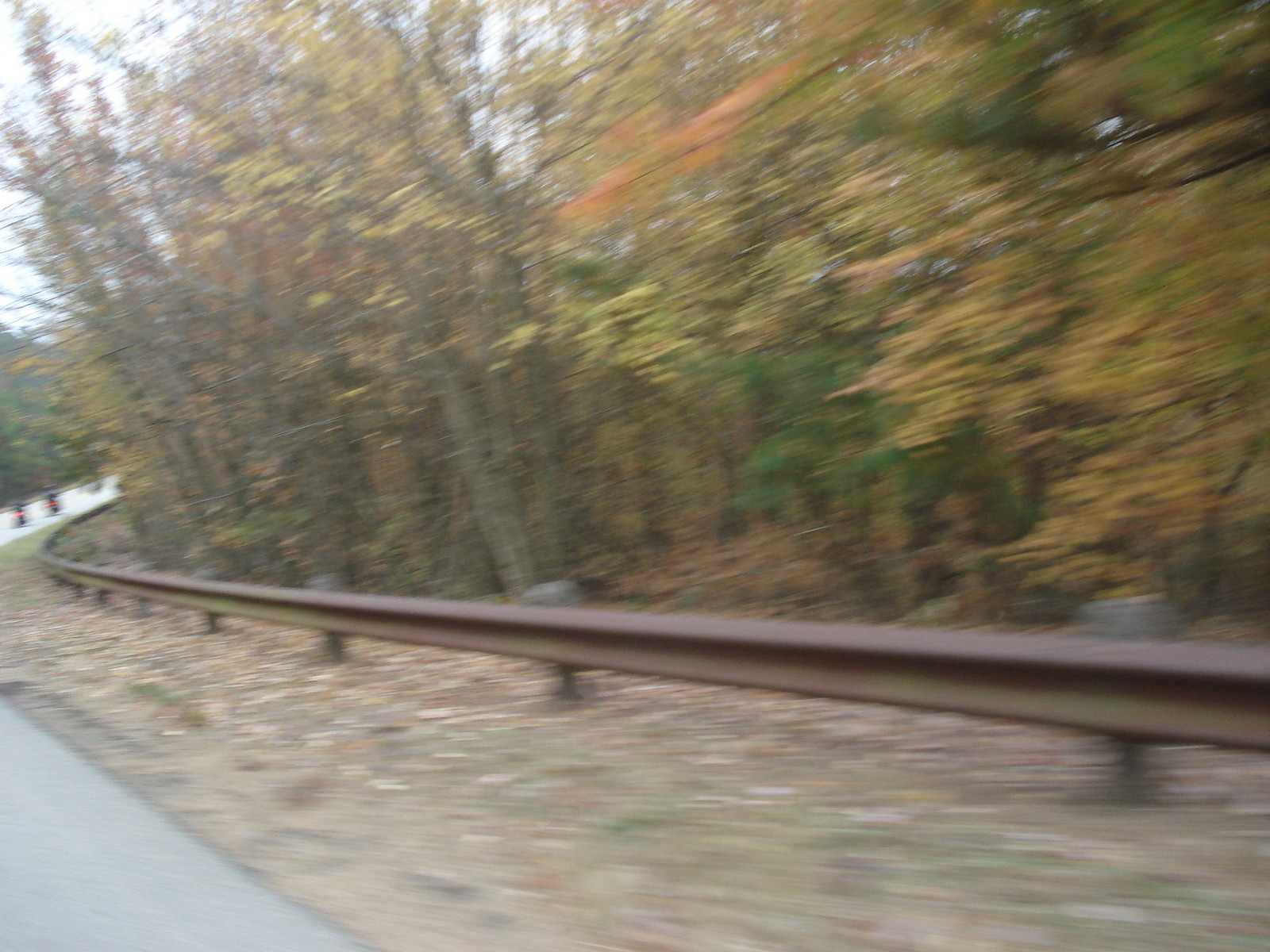A blurry photograph taken from inside a moving car captures the shoulder of a winding highway or country road. The light-gray pavement of the road curves from the bottom left corner to the top left corner of the image. Adjacent to the road is a dirt shoulder scattered with fallen autumn leaves. A brown metal railing follows the curve of the road, separating it from a dense forest. In the background, the forest features trees with thin trunks and foliage in vibrant shades of green, yellow, and orange, highlighting the seasonal transition to autumn.